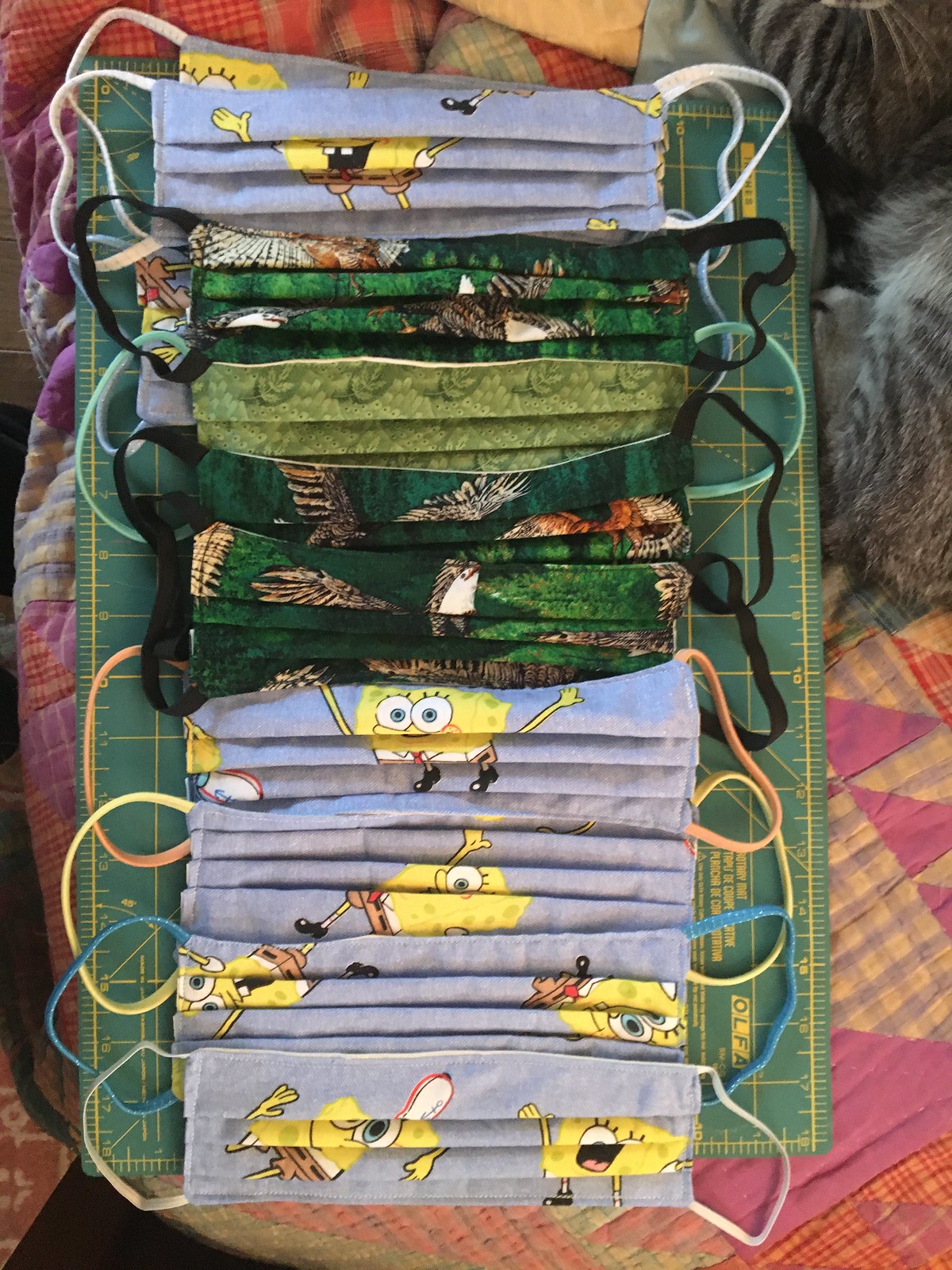A photograph depicts ten folded cloth masks arranged on a dark green grid mat with yellow measurements, atop a colorful, multi-patched quilt-style comforter. The masks, which are commonly used for COVID-19 protection, feature two distinct patterns. Five masks display a cheerful SpongeBob with his arms spread wide against a soft gray-blue background, and the other five have a green backdrop adorned with butterflies in flight. The intricate butterfly patterns are somewhat obscured due to the folds. Positioned in the top right corner, a gray cat with darker stripes can be seen partially curled up. The vibrant bedspread beneath adds a patchwork of calico colors, enhancing the lively atmosphere of the scene.